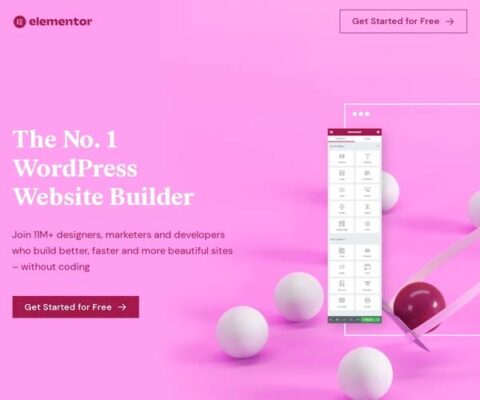This is a screenshot from an email website featuring a promotional banner for Elementor, a WordPress website builder. At the top, "ELEMENTOR" is prominently displayed in dark red, lowercase letters. Below this, a prominent pink rectangle contains the call-to-action button "Get Started for Free," accompanied by a right-pointing arrow.

The background of the banner is a vibrant pink, creating a visually striking contrast. On the left side of the banner, the text reads: "The Number One WordPress Website Builder. Join 11 million+ designers, marketers, and developers who build better, faster, and more beautiful sites without coding." Below this text, a red rectangle repeats the call-to-action, "Get Started for Free," again with a right-pointing arrow for emphasis.

To the right side of the text, there is an image featuring a pop-up window with text that is too small to read. This image includes five white balls and one red ball, adding a visual element to the banner.

The image is purely graphical, with no depictions of people, animals, birds, plants, flowers, trees, buildings, automobiles, airplanes, or helicopters.